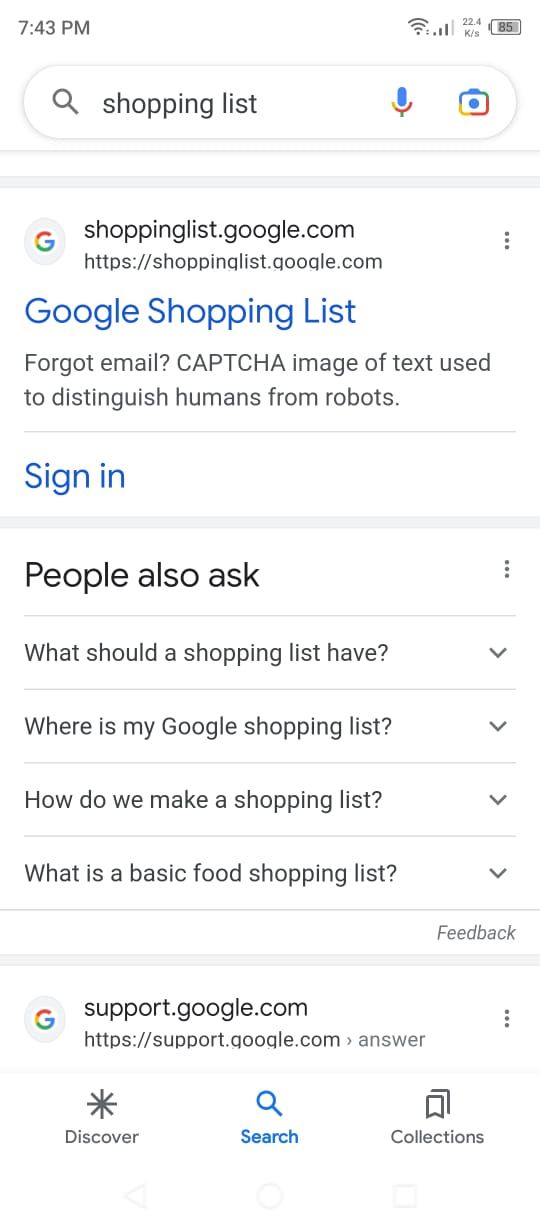The image depicts a screenshot of a webpage with a white background. At the top of the page, the time "7:43 p.m." is displayed. Below the time, there is a search bar with the text "shopping list" entered. The search bar has a microphone icon next to it. Below the search bar, a blue and red box with blue text inside it is displayed.

Further down, there are a few lines of text accompanied by the Google "G" logo, which is in red, yellow, and blue. The text reads "shoppinglist.google.com" followed by "Google Shopping List." There is a prompt to "forgot email," and an instruction to "capture image of text used to distinguish humans from robots." On the right side of this section, three vertical dots are visible.

Next, there's a sign-in button highlighted in blue. Below the sign-in button, there is a box labeled "People also ask," featuring a series of questions with down arrows next to them. The questions are:
1. "What should a shopping list have?"
2. "Where is my Google shopping list?"
3. "How do we make a shopping list?"
4. "What is a basic food shopping list?"

Below these questions, the text "Feedback" is displayed along with a blue line underneath it. Finally, there is the Google "G" logo inside a circle, with the text "support.google.com" next to it, followed by three vertical dots. At the bottom of the image are the options "Discover," "Search," and "Collections."